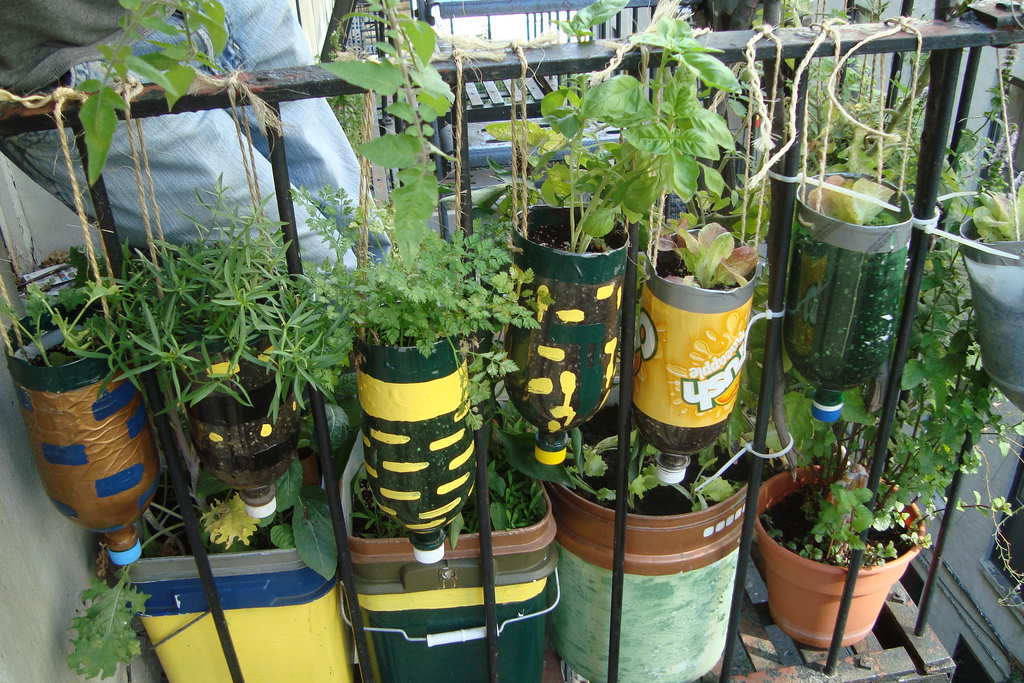The image depicts an urban balcony with wrought iron railings adorned with several inverted two-liter soda bottles repurposed as flower pots. Each bottle, some of which retain their original logos while others are painted with white stripes, hangs from twine and is filled with soil, nurturing a variety of plants. Below these hanging pots, the balcony supports a makeshift garden featuring assorted plastic totes and buckets in various colors—yellow, black, green, and reddish-brown—all brimming with additional greenery. The scene captures the creativity in urban gardening, highlighting the use of recycled materials to cultivate plant life in a small outdoor space. The photo is taken during the daytime, and a person in jeans can be seen standing behind the railing to the left.